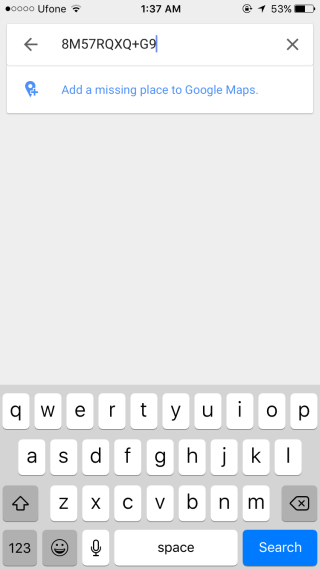The image depicts a vertical phone screen with a gray background, roughly two and a half times taller than it is wide. At the top of the screen, the status bar displays various normal phone settings: the carrier name "you phone" on the upper left, signal strength bars, the time "1:37 AM" in the center, and a battery indicator at 53% on the upper right, alongside other standard icons.

Below the status bar are two horizontal white boxes. In the first box, there is a left-pointing arrow on the left side, a string of random characters "8M57RQXQ + G9" in the center, and an 'X' symbol on the right side. The second box is blue and features a pin icon with a plus sign in the lower right-hand corner, positioned on the left side of the box. To the right of this icon, text reads "Add a missing place to Google Maps."

The remainder of the viewing area is filled with the gray background. At the very bottom of the screen, occupying about the lower third of the image, is a standard QWERTY keyboard layout.